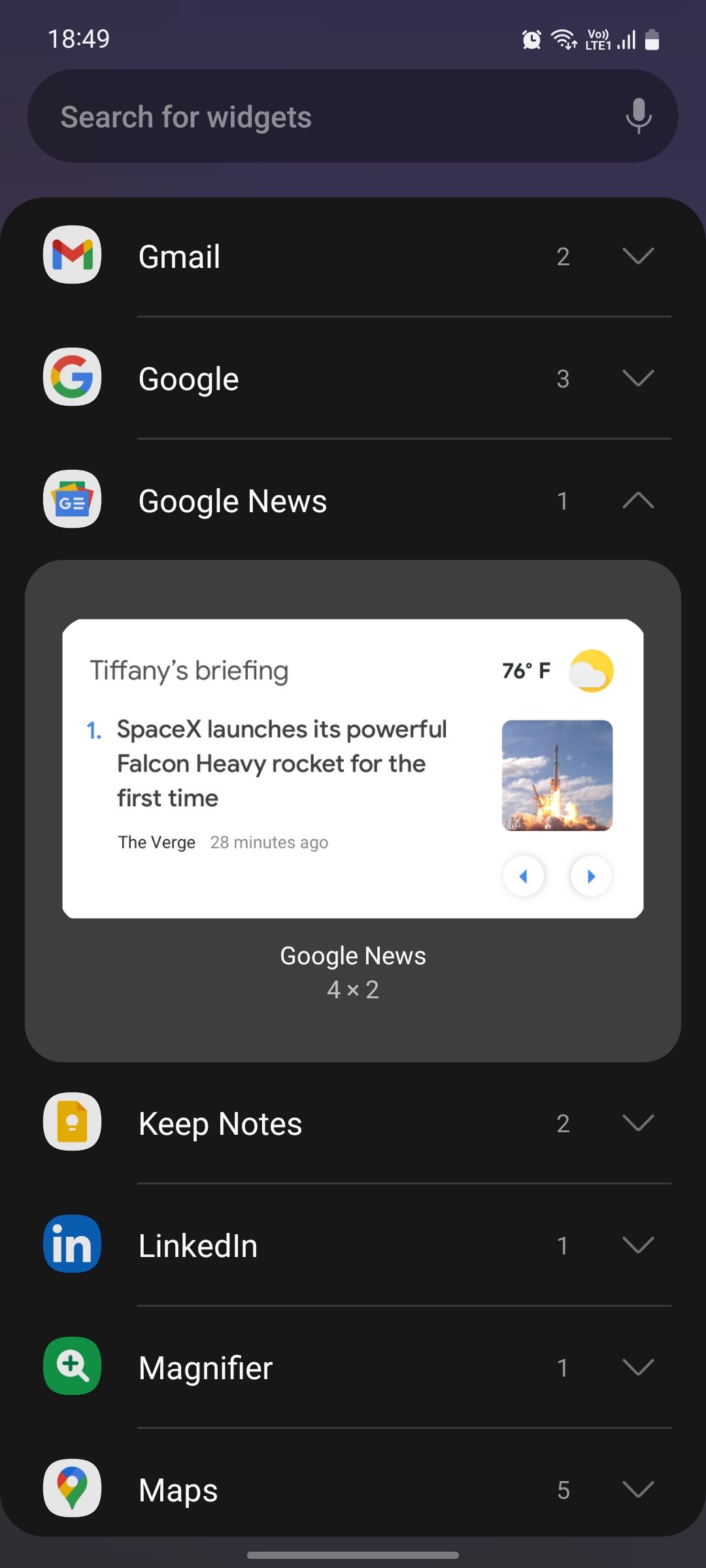This is a detailed screenshot from a phone displaying the time 18:49 with approximately half a battery charge. The interface features a search box with the text "Search for widgets" alongside a microphone icon set against a purplish background transitioning to a black background below. Beneath the search bar are several labeled icons, arranged vertically, which include Gmail, Google, Google News, Keep Notes, LinkedIn, Magnifier, and Maps, each accompanied by respective numerical notifications: 2, 3, 1, 2, 1, 1, and 5. Parts of the list are obscured by a pop-up notification titled "Tiffany Briefing," highlighting news from The Verge about SpaceX launching its powerful Falcon Heavy rocket for the first time. The current temperature is displayed as 76 degrees Fahrenheit and partly cloudy. The notification includes an image of the spaceship taking off from the launch pad and is labeled "Google News 4x2" at the bottom.